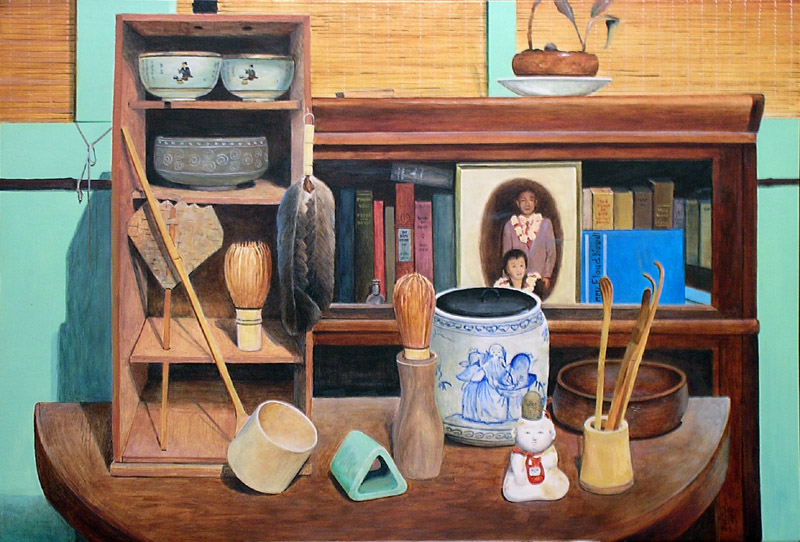The image is a highly realistic drawing of a scene set inside an Asian person's home, featuring detailed elements and artifacts. The focus is a half-moon brown wooden table positioned against a green wall with thin horizontal bamboo slats covering the windows. On the table, there is a four-level shelf that holds a variety of items including two teacups, a bowl with kitchen utensils, and a shaving brush. Resting on the shelf is also a pipe, a long stick attached to a cup, and another brush. Adjacent to the table is a brown wooden bookshelf containing books and a photograph of an Asian couple, where the man is standing and the woman is sitting in front of him. Atop the bookshelf is a white saucer with a brown pot, from which a plant is growing. The overall composition of the drawing captures a combination of daily life and cultural elements, showcasing various implements that suggest a blend of kitchen and personal grooming tools.